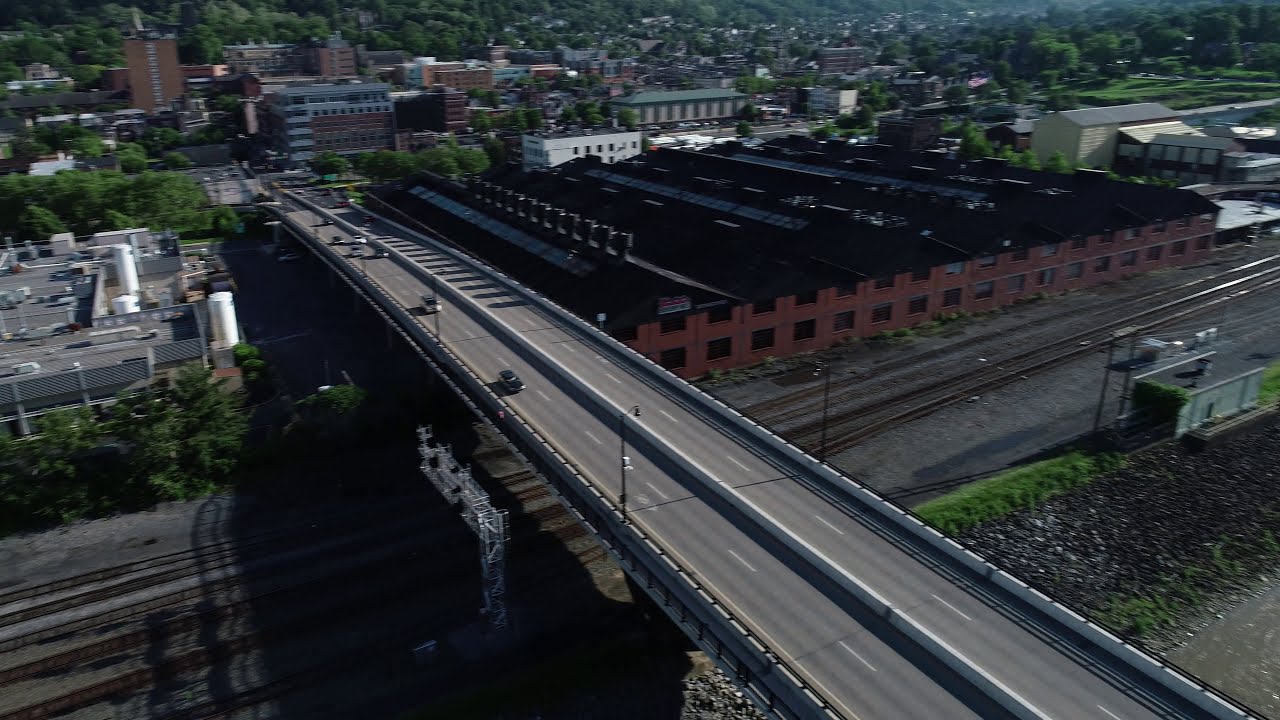The photograph captures a long freeway overpass with a four-lane highway, consisting of two lanes in each direction, leading into a densely-packed cityscape. The bridge is bordered by white cement barriers on both sides and a similar barrier running along the center median. It stretches over a set of train tracks that are slightly recessed into the ground, casting a shadow over them. On the right side of the bridge, just in front of the railroad tracks, stands a large, two-story brick building with an orange facade and a black roof, resembling a commercial warehouse. Sparse trees, full of lush green foliage, are interspersed among the city buildings, creating a mix of urban architecture and natural elements. The city in the distance is characterized by a variety of commercial buildings of different heights and colors, contributing to a vibrant metropolitan skyline. A few cars are visible on the freeway, traversing the overpass that slopes gently downwards as it approaches the urban area.